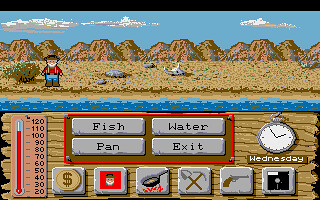The image appears to be a screenshot from a video game designed for a TV screen. The upper part of the screen showcases an Arizona desert landscape, characterized by a clear blue sky with scattered clouds, high hills in the background, and a vast flat plain in the foreground. On the left side of this scene, there's a small bush. A bearded man wearing a wide-brimmed hat, a long-sleeved red shirt, blue pants, and high boots stands amidst a couple of scattered rocks on the plain. A stream of water runs across the landscape.

The lower half of the screen displays the game's user interface. On the left side, there's a thermometer with a maximum reading of 120, currently indicating a temperature of about 105. Below the thermometer are four square gray buttons encased in a red outline box, which sits on a brown background. The buttons are labeled "Fish," "Water," "Pan" (below "Fish"), and "Exit" (below "Water").

On the right side, there's an old-fashioned timer set to approximately five minutes to 2, with "Wednesday" displayed just below it. Beneath the day indicator are six more gray buttons. From left to right, these buttons feature icons of a dollar sign, a man's face, a flaming frying pan, crossed pickaxes, a gun, and a save disk. This entire interface section is set against a wood-textured background, enhancing the rustic theme of the game.